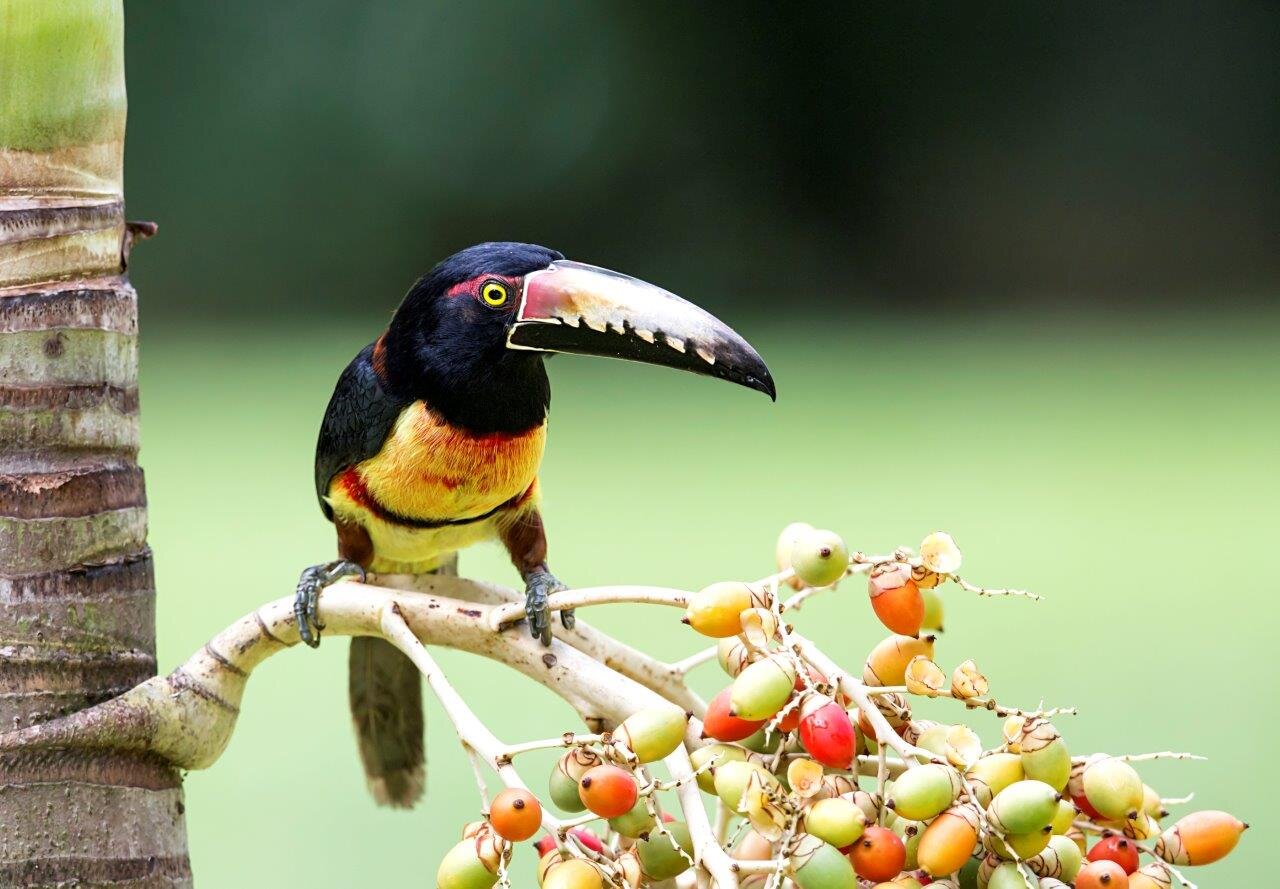In this detailed photograph, a striking toucan is perched on a branch extending from the left side of the frame toward the bottom right. The bird is positioned slightly off-center to the left, gazing directly at the camera with its prominently green eye encircled by a red stripe. Its head sports a dark indigo hue, transitioning to a mostly black upper body. The toucan's large, distinctive beak displays a gradient: light-colored on top with tinges of red near the face and darkening towards the tip, while the lower part is entirely black. The chest of the bird is vibrant yellow, accentuated by a black and red band midway down. Beneath its sturdy brown legs are black feet, and its tail extends directly behind, tinged in a grayish shade.

The branch the toucan perches on is white, sprouting from a tree which resembles a palm with a green trunk and horizontal, brown ridges. Adorning the branch are clusters of assorted berries in striking hues of red, orange, green, and yellow, adding a burst of color to the scene. The background is a soft blur of various shades of green, indicating a lush, tropical setting. This out-of-focus backdrop ensures the toucan and the vivid berries remain the focal points of the image, accentuating the bird's majestic presence and the vibrant environment it inhabits. It looks as though the toucan might be poised to feast on the abundant berries surrounding it.